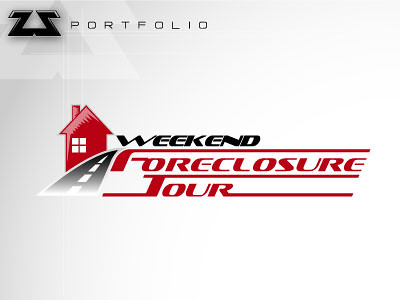The image features a small graphic that resembles a title slide from a presentation, set against a light gray to white gradient background, with the bottom right corner appearing white and the gradient transitioning to light gray towards the left and top. In the top left corner, there's a logo consisting of two black 'Z' letters mirrored back-to-back, followed by the word "Portfolio" in thin black text. Central to the graphic is a stylized depiction of a red house with a single window and a chimney, adjacent to a gray-to-black road with dashed white lines. The text "Weekend" is rendered in black above the words "Foreclosure Tour" in red, with notable decorative extensions on the letters 'F', 'T', and 'R'.